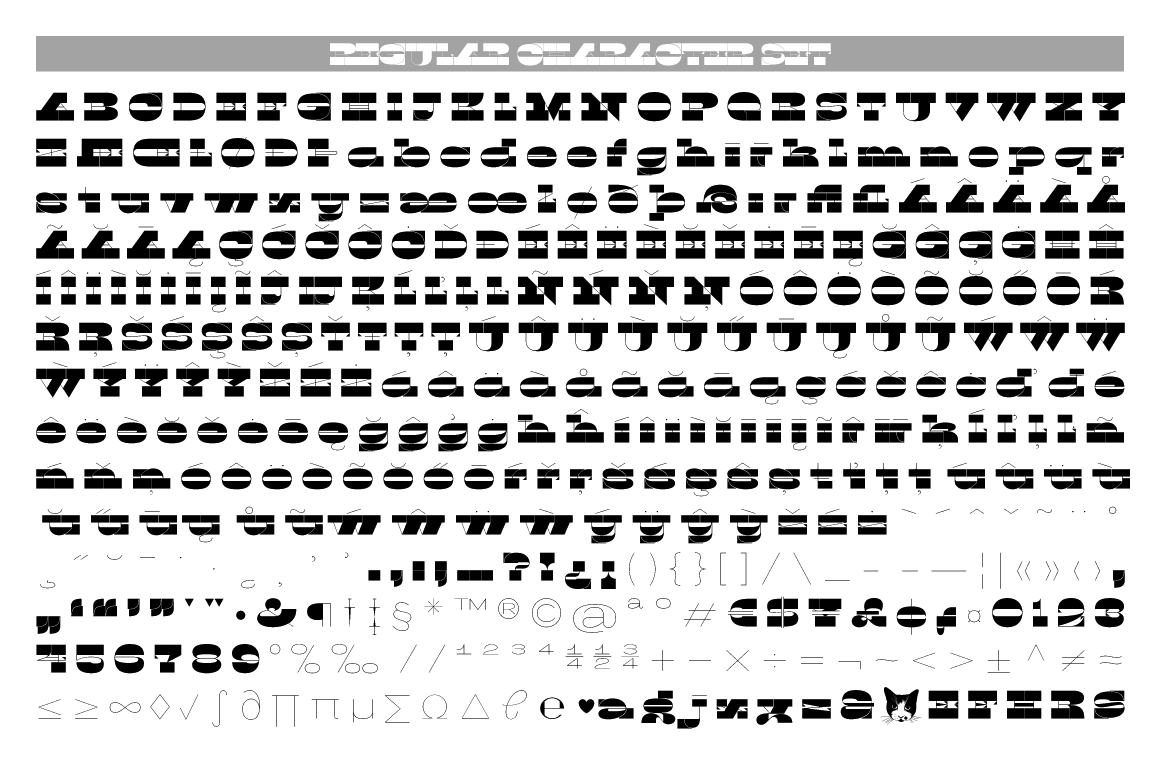This image features a comprehensive chart displaying various stylized characters and symbols. The top section, in gray with white lettering, is difficult to read but appears to organize the content into categories. Below, the chart displays the entire alphabet from A to Z, each letter rendered in a variety of artistic styles across approximately 14 rows.

The characters include unique and fancy versions of standard letters, which are not typically found on a standard keyboard. Scanning towards the bottom, the chart showcases more intricate symbols. Specifically, the last three rows exhibit unusual and decorative representations of double or triple 'S's, an assortment of hand-drawn symbols such as an asterisk, a "TM" symbol, a registered trademark "R", a copyright "C", and an "@" symbol. 

Additionally, there are hand-drawn percentages, numeric characters including floating versions of 1, 2, 3, and 4, and fractions like 1/4, 1/2, and 3/4. Unique to this collection, a whimsical touch is added with a random burger and cat emoji at the bottom, along with some Middle Eastern-looking flags, further broadening the assortment of characters available. This chart appears to be a resource for inserting special characters that aren't accessible through standard keyboard input, providing a diverse range of symbols for various uses.